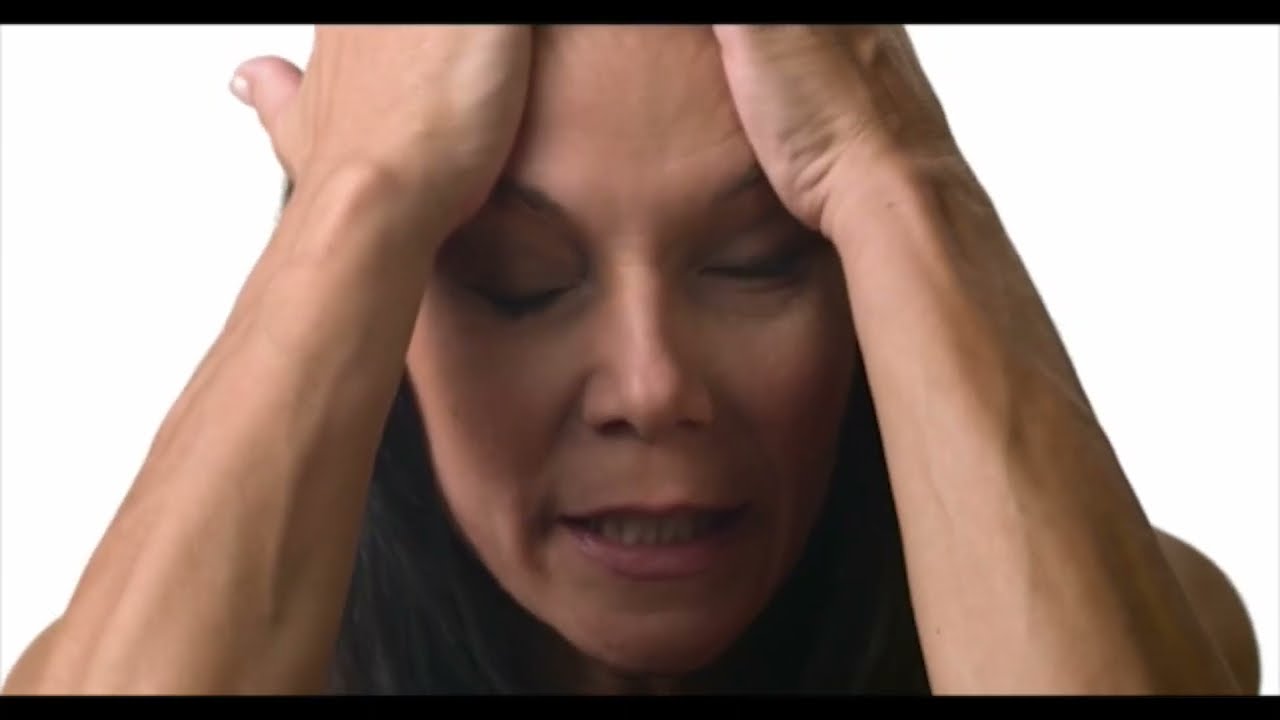This is a detailed photograph of a woman, possibly a white or Latina female, with dark brown hair cascading slightly forward on both sides of her face. Her eyes are closed, and she appears to be experiencing significant discomfort, stress, or fatigue. Her mouth is slightly open, with her teeth showing, conveying an impression of pain or exhaustion. Both of her hands are pressed against her forehead, applying pressure and pulling her eyebrows upward. The veins in her arms are prominently visible, suggesting tension. Her elbows and arms seem to be resting on a surface, and she is wearing a tank top, as indicated by the visibility of her shoulder. The background of the photo is stark white, emphasizing the woman's distressed expression and posture.